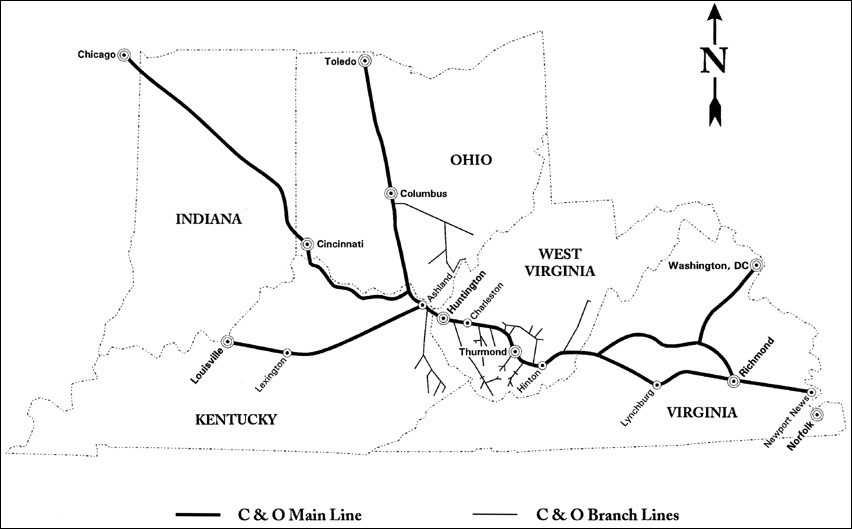The image is a detailed black and white map specifically highlighting the states of Indiana, Ohio, Kentucky, West Virginia, and Virginia. At the top right, there's an arrow marked with an "N" indicating that north is up. The map features bordered lines in black and lighter gray to represent different railway lines: a thick, black line for the C&O main line, and a thinner, gray line for the C&O branch line. The C&O main line stretches from Chicago, Illinois, moving southeast through major cities, including Toledo, Columbus, Cincinnati, Louisville, Washington D.C., Richmond, and finally reaching Norfolk, Virginia. The branch lines mainly traverse through Ohio, West Virginia, and Kentucky, connecting various smaller towns and cities. The map provides a visual illustration of these railway routes, indicating how they interconnect and span across these five states.